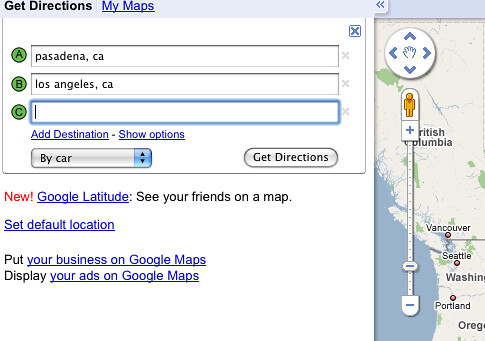The screenshot displays a Google Maps interface with the following details: 

At the top bar, the options "Get Directions" and "My Maps" are prominently labeled. Below this, there are three input lines for destinations: Line A shows several green dots and reads "Pasadena, CA," Line B reads "Los Angeles, CA," and Line C is blank. Below these lines, in blue lettering, it reads "Add Destination - Show Options."

To the side, there is a capsule-shaped button with a blue background labeled "By Car" with up and down arrows next to it. Adjacent to this capsule, on the right, is another capsule labeled "Get Directions." Beneath this, there are four text prompts:
1. "New Google Latitude - See Your Friends on a Map."
2. "Set Default Location."
3. "Put Your Business on Google Maps."
4. "Display Your Ads on Google Maps."

On the right quarter of the screenshot, there is a vertical map starting from British Columbia at the top, followed by Vancouver, Seattle, Washington, and finally Portland, Oregon. This section includes a ruler-like measurement tool with a plus and minus sign.